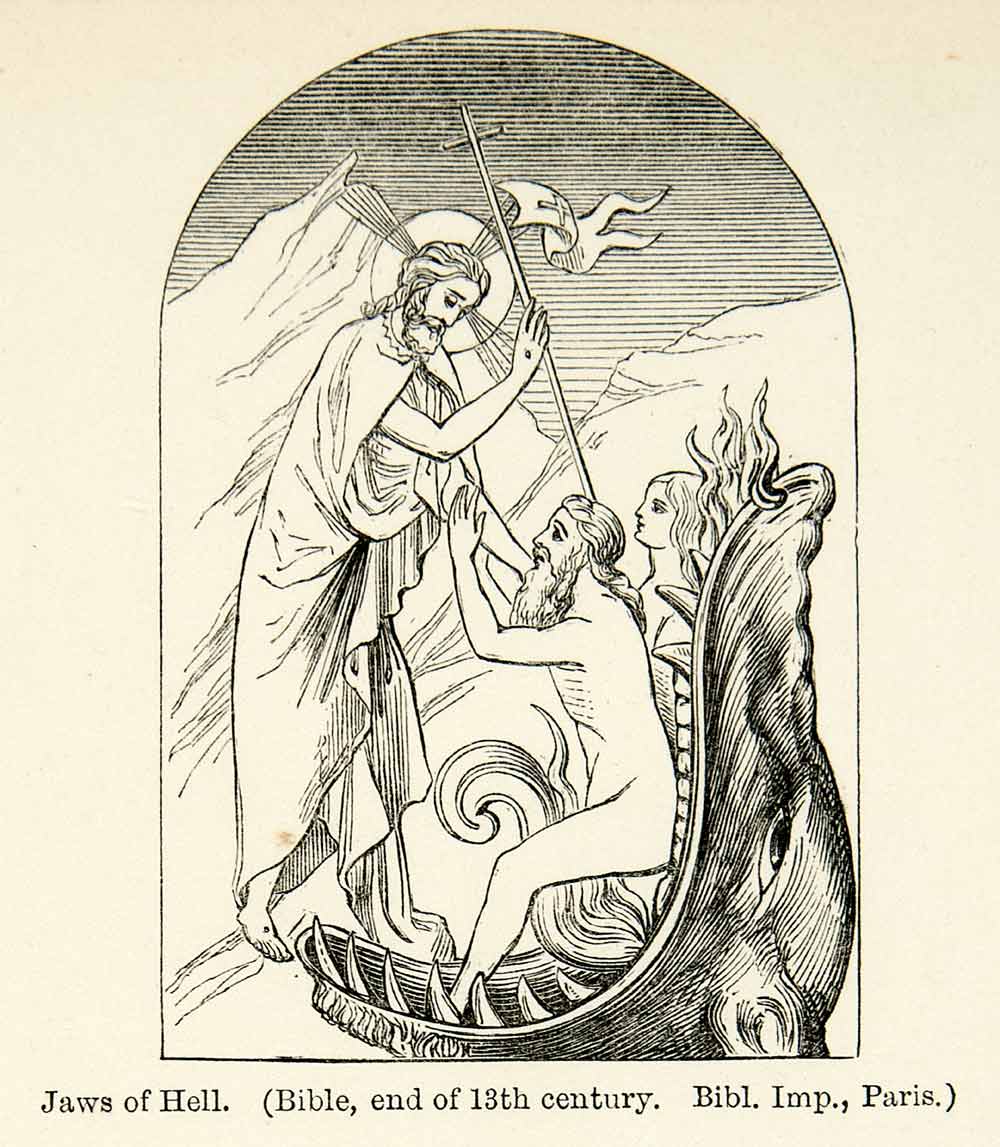The image, set on a cream-colored background resembling aged, yellowed paper, depicts a detailed black and white drawing within a tombstone-shaped frame. The composition centers around a religious scene titled "Jaws of Hell, Bible, end of 13th century, B-I-B-L. I-M-P., Paris." In the foreground, a robed and haloed figure, likely Jesus, stands with a long cross in his right hand, looking downward. This figure has a distinctive halo with lines pointing in a cross shape. He places his hand on the shoulder of a bearded, long-haired naked man who sits within the menacing jaws of a wolf or dragon-like creature, characterized by sharp teeth and a gaping mouth. The man, along with a naked woman beside him, are seemingly trapped inside this monstrous mouth. Behind them, the creature's torso and head rise ominously. In the background, black horizontal stripes represent the sky, underlined by distant mountains. This evocative scene captures a dramatic moment of confrontation and entrapment, rich with religious and mythical symbolism.